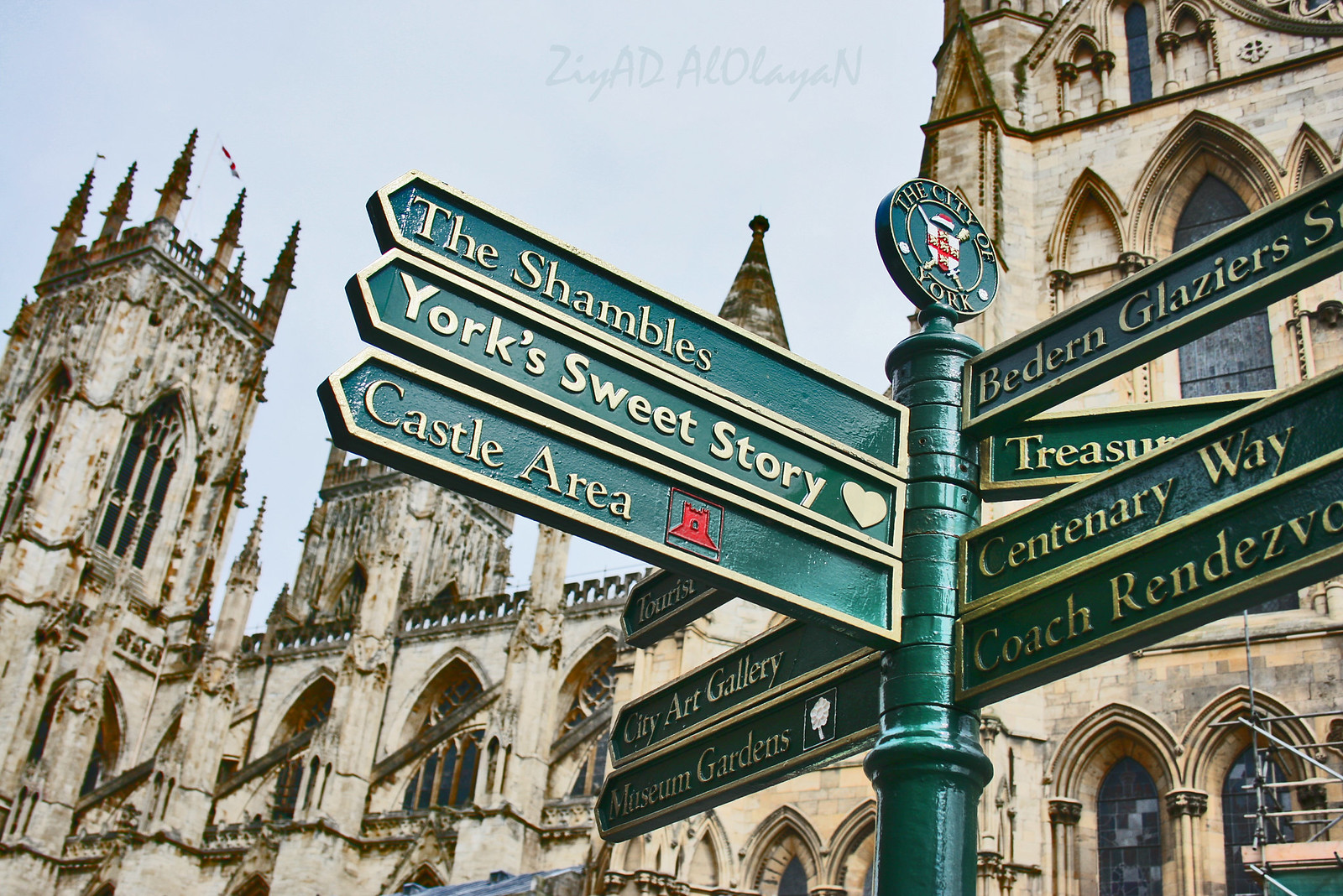This daytime landscape photograph captures a bustling intersection in a European city, with the majestic backdrop of a medieval castle. The castle's gothic architecture is highlighted by its towering spires, arching windows, and flag-topped turrets, creating an aura of ancient grandeur. In the foreground stands a large, green street sign adorned with intricately detailed gold lettering and various directional arrows, indicative of the city's historical significance and tourist attractions. Prominent directions include 'The Shambles,' 'York's Sweet Story,' 'Castle Area,' identified by their respective logos—a white heart and a red castle. Additional markers, like 'Bedern Glaciers,' 'Centenary Way,' and 'Coach Rendezvous,' suggest the city's rich network of pathways and points of interest. The sign also features a circular emblem at the top, reading 'City of York' with a shield logo, grounding the scene firmly in its historical context. The overall style of the photograph is representational realism, capturing the ornate details and the intersection’s dynamic layout.